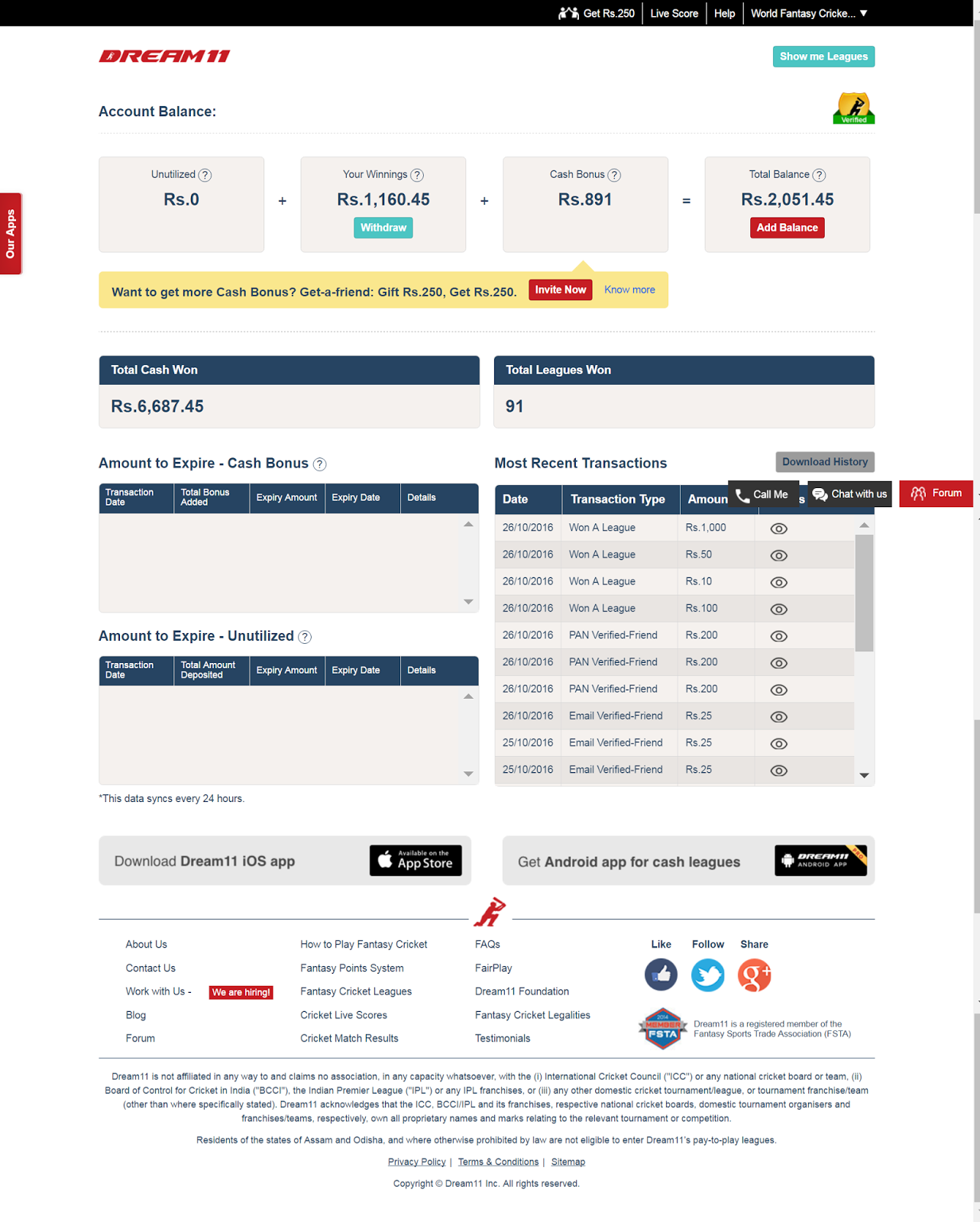This screenshot captures a detailed view of the financial dashboard for a user on the website Dream11, a platform centered around fantasy sports. Prominent features of the interface indicate that it deals with financial transactions in Indian Rupees (Rs). At the top of the screen, there are navigation options including 'Live Score', 'Help', 'World Fantasy', and 'Show Me Leagues'.

The user's financial summary is displayed with the following details:
- Account Balance: Rs. 0
- Winnings: Rs. 1160
- Cash Bonus: Rs. 891
- Total Balance: Rs. 2051
- Total Won: Rs. 6687
- Leagues Participated: 91

The recent transaction history from 2016 shows the user has made multiple withdrawals from various sources:
- From 'WannaLeague'
- From 'Pan Verified Friend'
- From 'Evil Verification'

Additionally, the interface promotes downloading apps related to the Cash League and provides a section for submitting Frequently Asked Questions (FAQs), comments, or questions. This comprehensive financial overview offers insightful details about the user's earnings, transactions, and participation on the Dream11 platform.